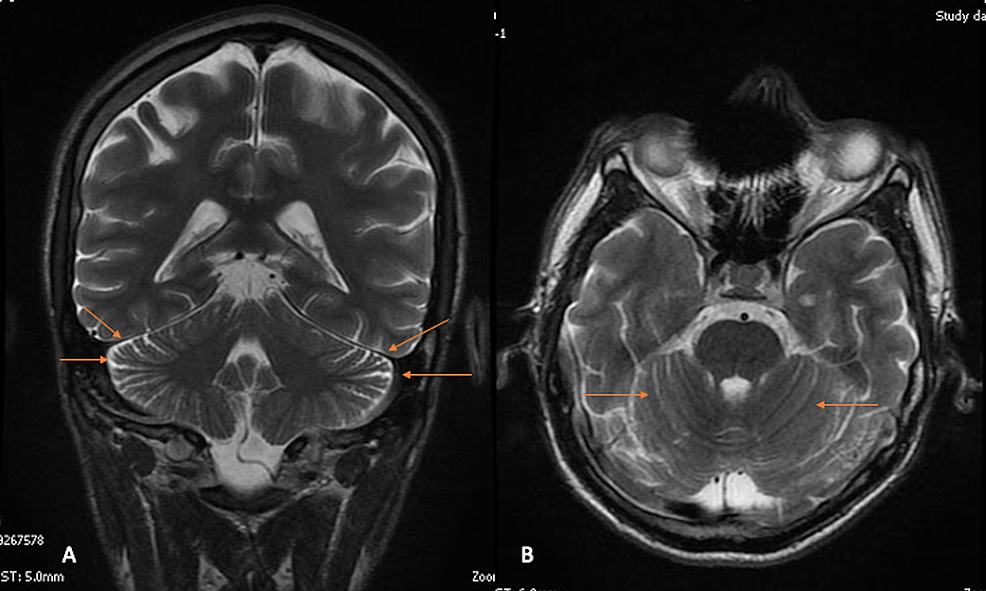This image displays two CAT scans of a brain, side-by-side against a black background, formatted in a landscape layout. The scan on the left seems to be taken from the back or front of the head, while the scan on the right appears to be from the top, looking down. Both scans feature orange arrows pointing to corresponding areas within each image. The image on the left shows an 'A' in the bottom left corner, while the right image has a 'B' in the same position. In addition to these letters, the bottom-left corner of both images contains the numbers '267578' followed by 'ST 5.0 mm', though part of the text is cut off. In the top right corner of both images, the word 'study' can be seen, partially cut off as 'DA', with the left image also displaying a 'negative one'. The scans are evidently of the same person's brain, taken from different angles and perspectives, providing a comprehensive view for diagnostic purposes.